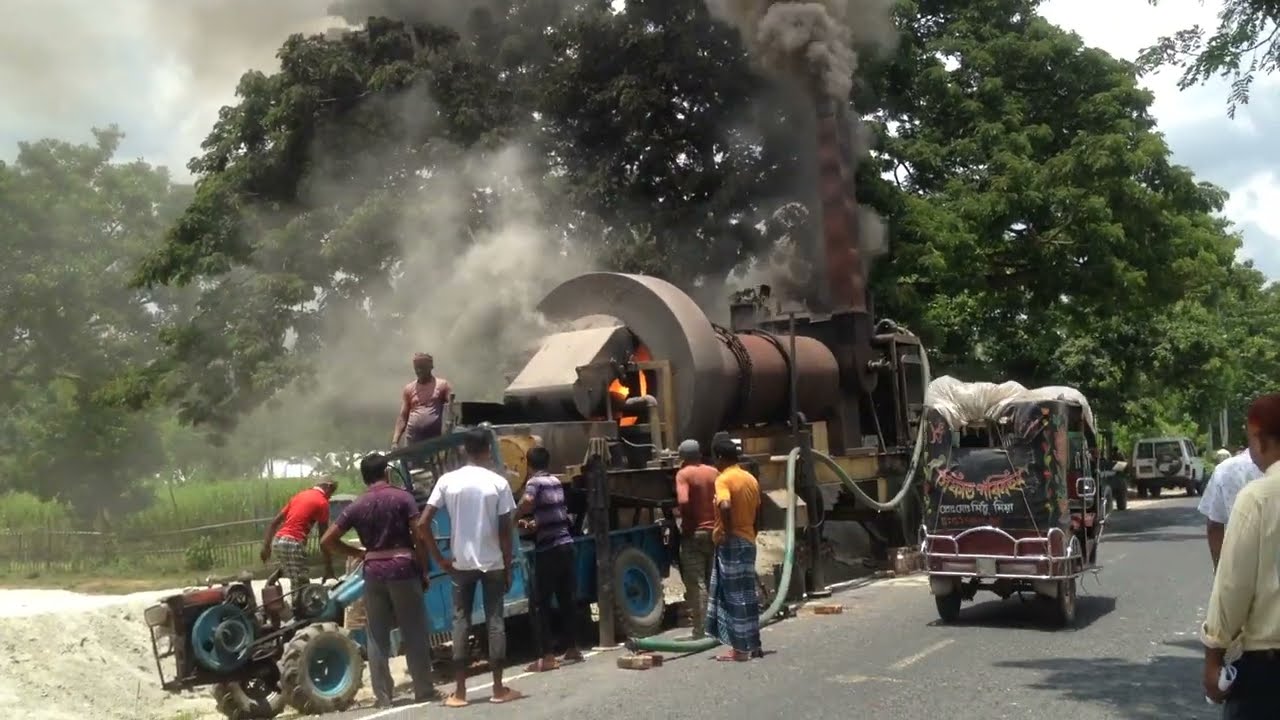The photograph captures a bustling scene on the side of a road where a large industrial vehicle, resembling a steam engine, is prominent in the center. The vehicle has a cylindrical top with a large gray end and a hose extending down its side. A significant amount of dark gray smoke billows from the smokestack, suggesting possible mechanical trouble or an accident.

Several African-American individuals surround the vehicle, appearing to work or inspect it closely. Two people, positioned at the back, face left while examining the equipment. Behind them, three more individuals stand alongside a blue wagon, looking intently forward. On a nearby platform, a person looks towards the vehicle and to the left, while another individual in a red shirt on the ground leans over, inspecting the right side. To the right of the main vehicle, a smaller cart or machine is also present, with two people nearby observing the scene.

In the background, the road extends into the distance where a vehicle travels in the opposite direction. A small fence and a large grassy area with trees flank the road on the left side, adding a touch of greenery to the otherwise mechanical and smoky tableau. The sky, filled with clouds, envelops the scene in a midday light, casting a grayish hue over the entire area. The mixture of white, gray, blue, green, red, yellow, orange, and tan colors punctuates various elements, contributing to the vivid depiction of this outdoor incident.